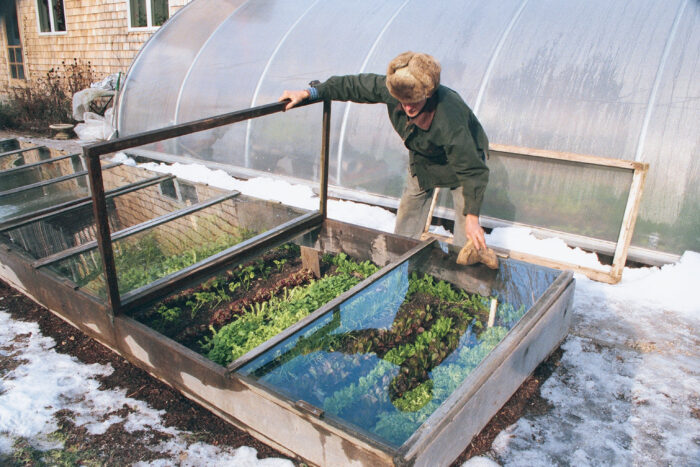In a cold, snow-dappled outdoor setting, a person, likely a man, is engaged in winter gardening. Dressed for the harsh climate in a deep olive green jacket, a fur hat with ear flaps, and grayish pants, he is bending over a series of encased garden beds. The man is carefully opening a glass hatch to inspect or tend to the verdant lettuce plants growing underneath. Adjacent glass panels stretch across the length of the garden, some of which are at ground level, while others appear below house level, possibly reflecting the nearby structures. Behind him stands a curved, pop-up greenhouse with condensation on the windows, alongside an unused panel leaning against it. In the distant background, a light-colored brick house with visible windows and front plants completes the wintry scene, illustrating a blend of nature and human ingenuity in an unforgiving climate.